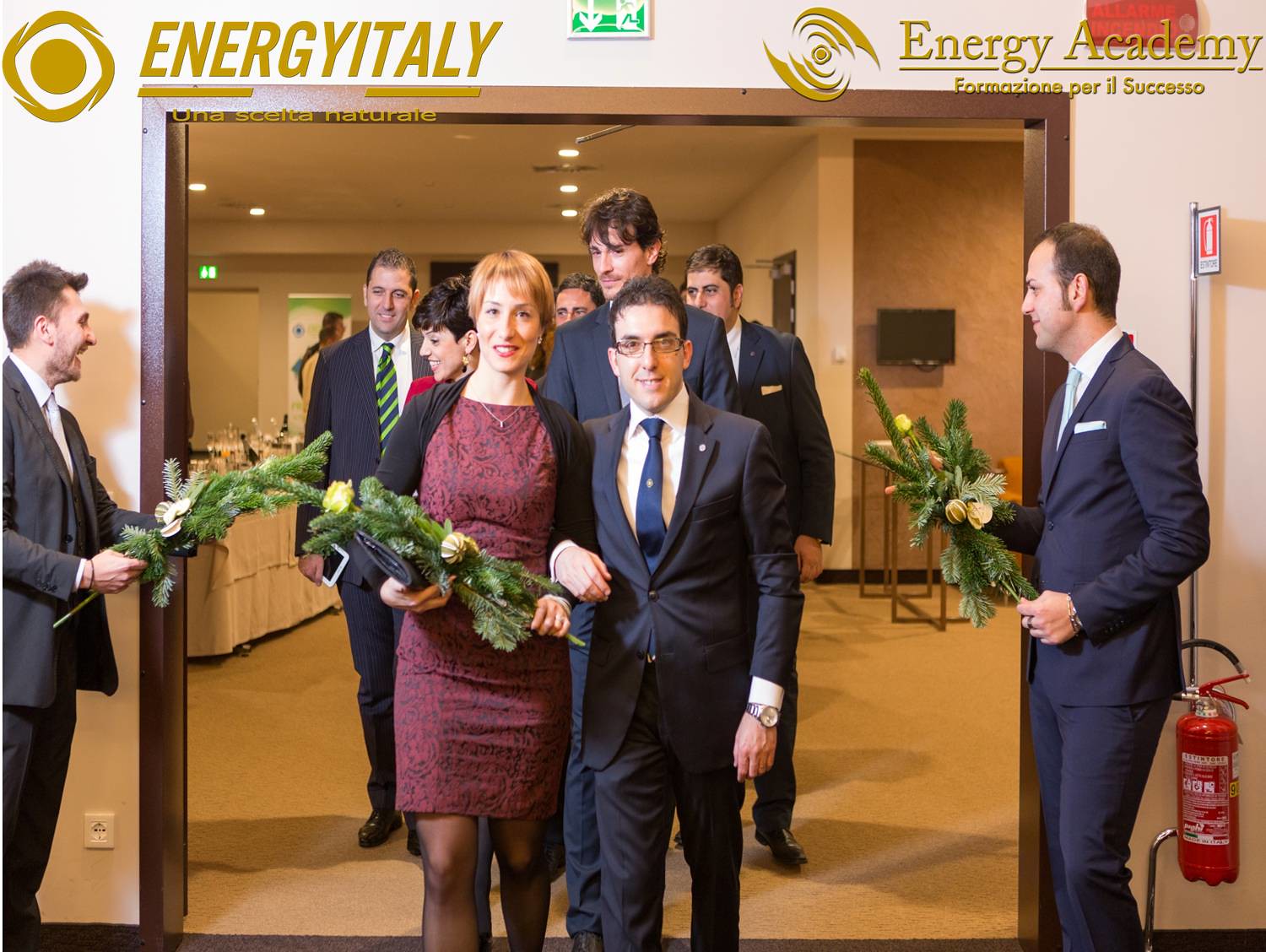In this detailed photo, a well-dressed group is seen exiting a room through an open pair of brown-framed double doors, presumably following a ceremony such as a wedding. At the forefront of the image, a tall blonde woman in a dark purple dress paired with a black sweater holds a long, green leafy arrangement in her left hand and a purse in her right. She is arm-in-arm with a shorter man, who sports a blue tie, a white button-down shirt under a blue suit, glasses, and a wristwatch. Both are smiling warmly at the camera.

Flanking the doorway, two men in dark suits hold out matching green leafy arrangements, creating an archway for the couple. Behind the leading pair, a crowd, consisting mostly of men in dark suits and ties, follows them out in a two-by-two formation. The surrounding indoor space features beige-colored walls and floors, adorned with a tan rug, a television displaying the phrases "Energy Italy" and "Energy Academy," and a piece of artwork. A fire extinguisher is also visible at the bottom of the scene.